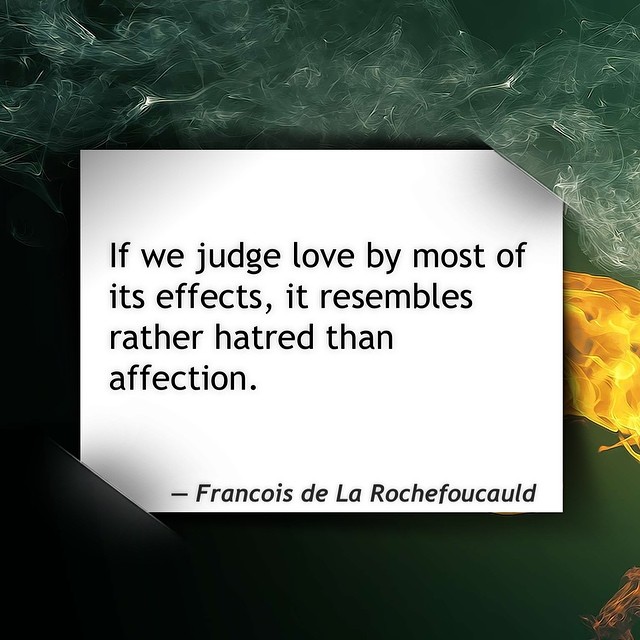The image showcases a white card positioned centrally within a decorative card holder. The card holder is predominantly dark green with a touch of yellow on the right-hand side, and it features a smoky white design at the top, accompanied by hints of orange. The card itself bears a dark gray print with an inspirational quote: "If we judge love by most of its effects, it resembles rather hatred than affection." At the bottom of the card, the quote is credited to François de la Rochefoucauld. The overall setup and style of the image suggest it's designed for sharing inspirational messages on social media.